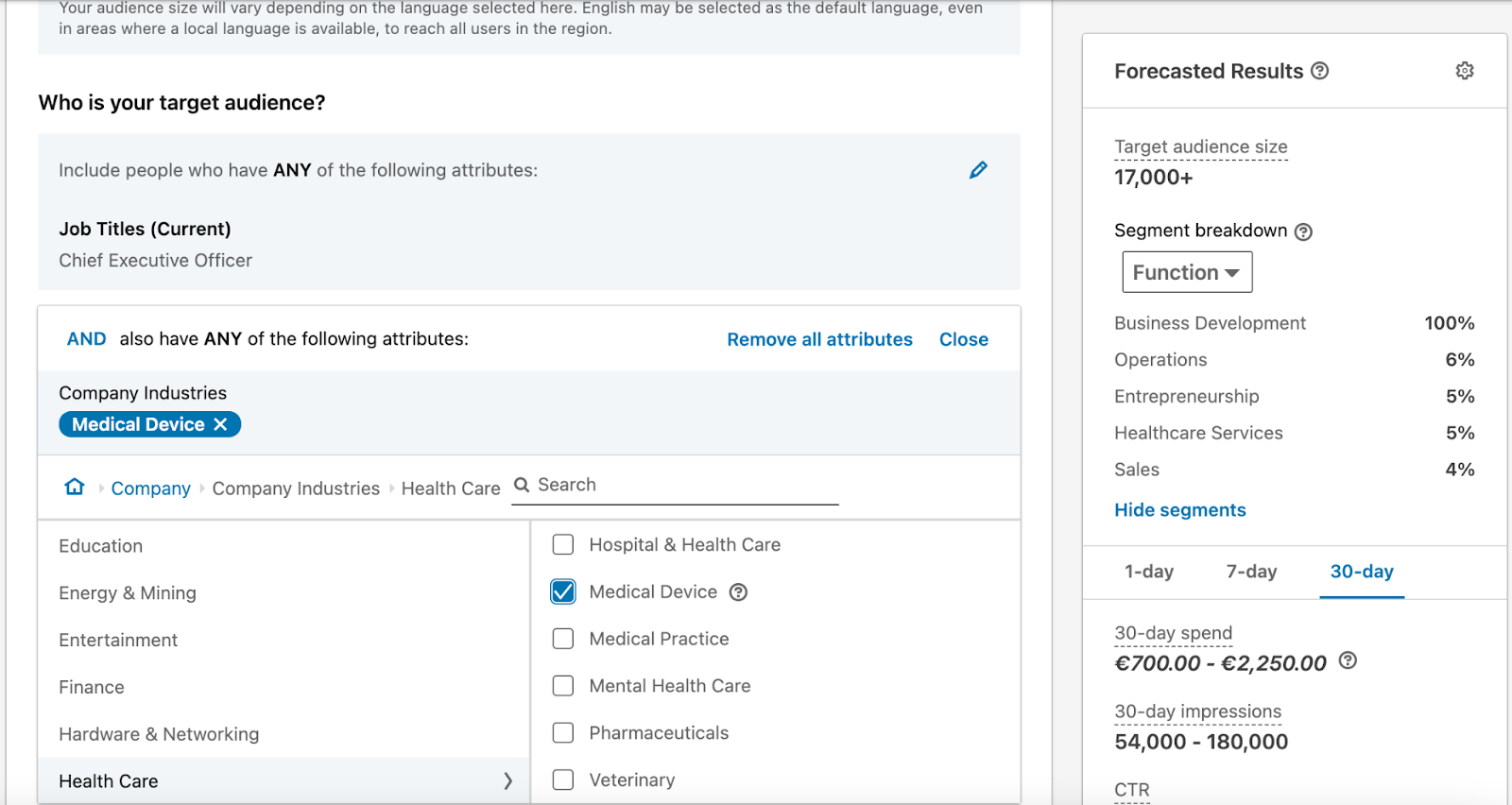Screenshot of an Administrative Marketing Configuration Page

This image is a partial screenshot of what appears to be an administrative interface for configuring marketing ads. The background of the interface is predominantly white.

At the very top of the image, a section is cut off but displays a light sky blue rectangle with a gray font message: "Your audience size will vary depending on the language selected here. English will be selected as the default language, even in areas where a local language is available to reach all users in the region."

Below this message, in bold black font, a query reads, "Who is your target audience?"

Directly underneath this question, there is another light blue rectangle. The content within mentions targeting individuals with specific attributes, starting with job titles. For instance, "Current: Chief Executive Officer" is listed.

Continuing below, it asks for additional attributes, displaying "Company industries." Here, "Medical Device" is highlighted in white font within a blue rectangle with rounded edges. It implies options exist for selecting various industries.

On the right side of the image, a long vertical white rectangle is dedicated to forecasted results. At the top of this section, accompanied by a question mark in a circle, it says "Forecasted Results."

Underneath this heading, it displays:

- "Target Audience Size": 17,000+
- "Segment Breakdown Function": Business Development, Operations, Entrepreneurship, Health Services, Sales. An option to "Hide Segments" is available in blue.

Options for ad durations are given, allowing selections of one day, seven days, or 30 days, with 30 days being selected in this instance. The "30-Day Spend" forecast is denoted in euros, ranging from 700 to 2,250 euros. Lastly, the "30-Day Impressions" estimate is provided, ranging from 54,000 to 180,000 impressions.

The screenshot captures a moment in the configuration process of a detailed and segmented ad setup in a marketing platform.